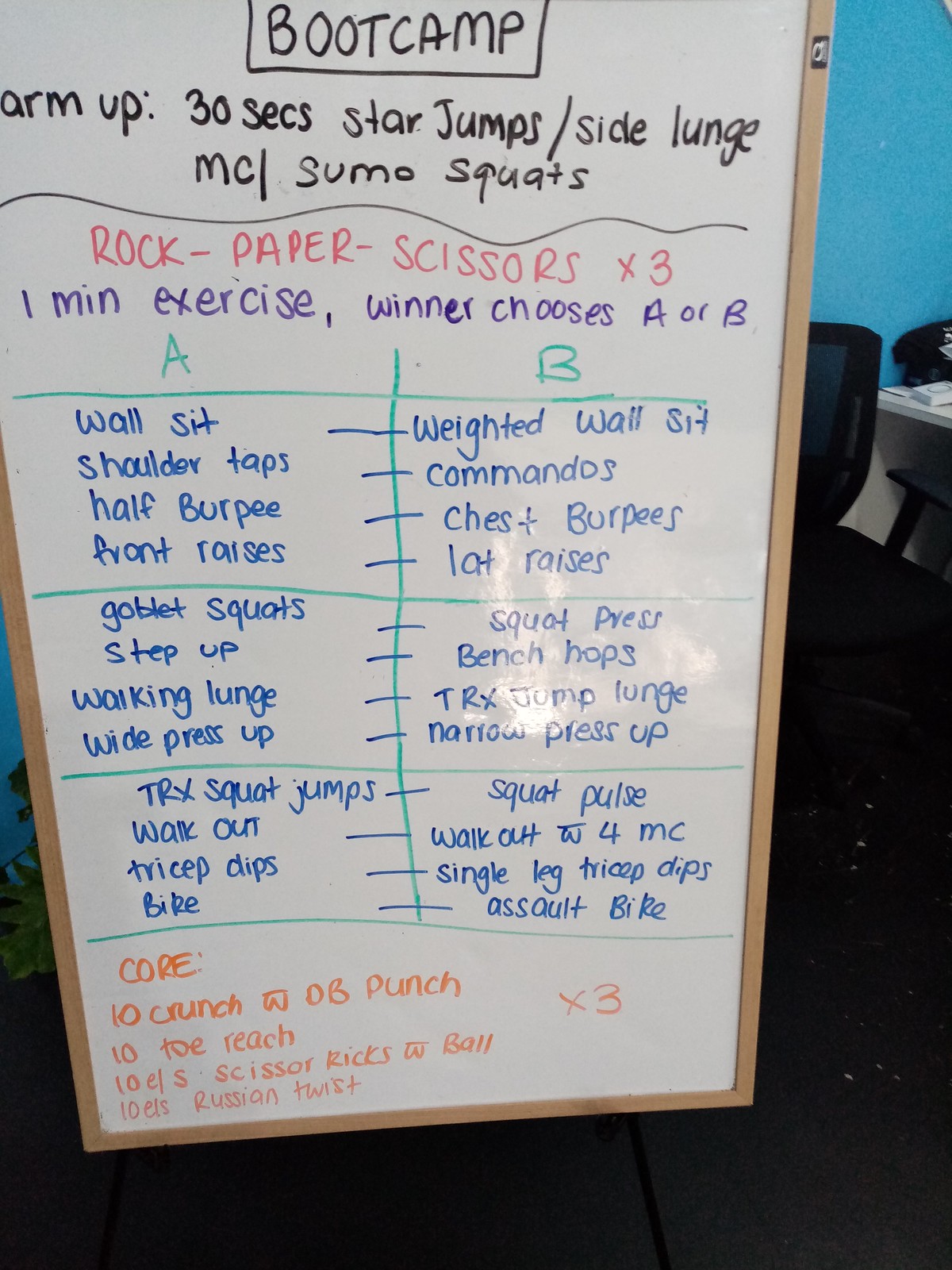The photograph captures a gym room featuring a prominent whiteboard with intricate workout instructions. The whiteboard, encased in a wooden border, is situated on a stand against a backdrop of blue walls and dark-colored office chairs. The floor is black, and a white table is visible. At the top of the whiteboard, "Bootcamp" is written inside a rectangular outline, followed by detailed warm-up instructions: 30 seconds each for star jumps and side lunges, and a sequence of exercises split between two columns labeled A and B. Column A lists: wall sit, shoulder taps, half burpees, front raises, goblet squats, step-ups, walking lunges, wide push-ups, TRX squat jumps, walkouts, tricep dips, and bike exercises. Column B includes: weighted wall sit, commandos, chest burpees, lat raises, squat press, bench hops, TRX jump lunges, narrow push-ups, squat pulses, walkouts, single-leg tricep dips, and assault bike sessions. The bottom section outlines core workouts in red: 10 crunches with dumbbell punches, 10 toe touches, 10 scissor kicks with a ball, and 10 Russian twists, with each set repeated three times.